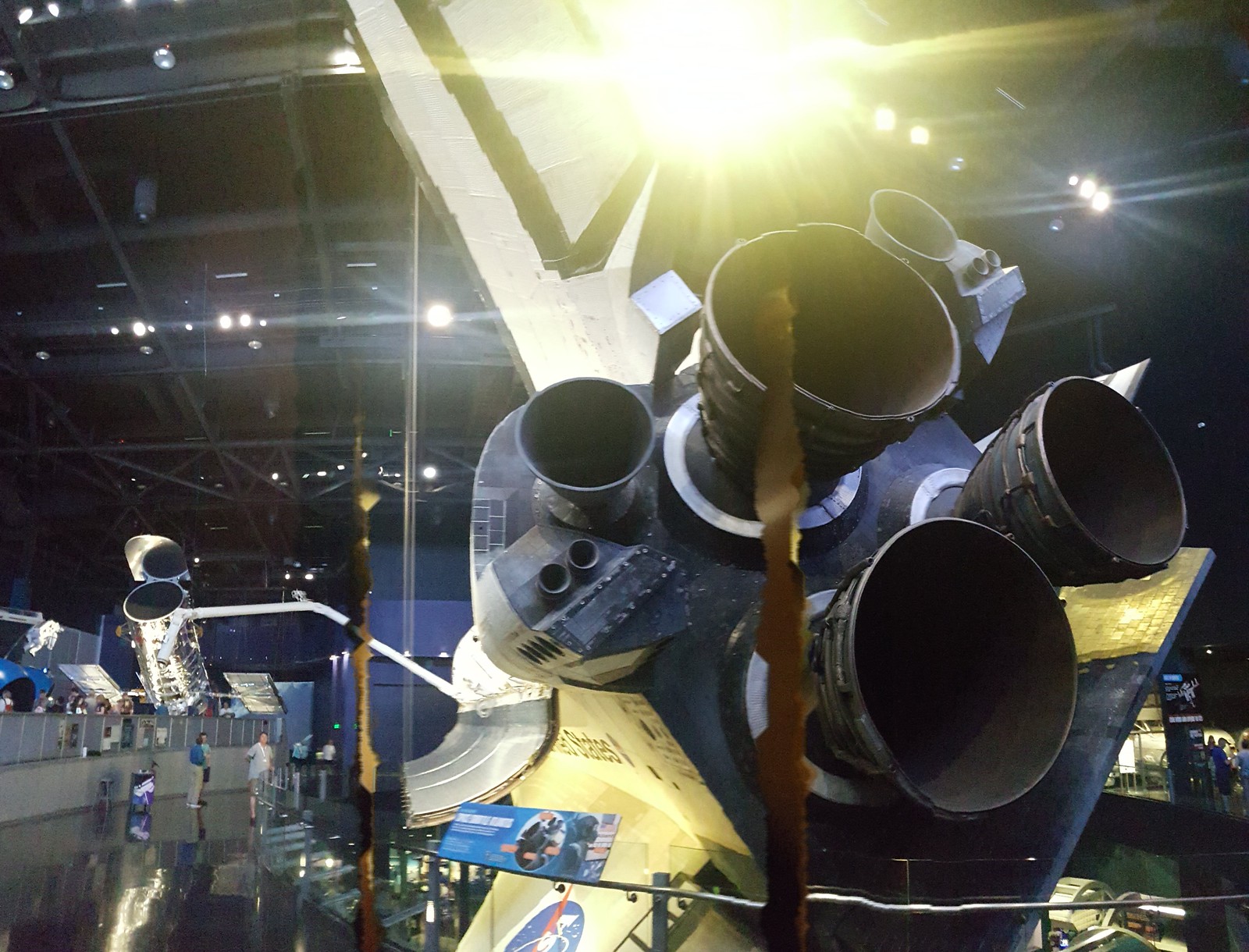The image depicts the expansive interior of a large, metallic-ceilinged building with an appearance suggestive of an air and space museum, possibly located in Florida or Washington, D.C. Bright white lights illuminate the space from the ceiling, which features an intricate arrangement of scaffolding or steel rafters. The glossy, dark blue or black floor reflects these lights, adding to the grandeur of the setting.

Dominating the foreground is the rear view of a space shuttle, its assemblage of conical jet engines—four or five in number—prominent and detailed. The shuttle angles forward slightly, with an articulated arm extending to hold a cylinder clad in a silvery material. Though there is some glare, the words “United States” are faintly visible on the side of the shuttle, indicating its identity.

In the bottom right corner, a group of people stands observing the exhibit, their attention focused on the shuttle and its accompanying informational plaques. The scene evokes a sense of admiration and curiosity as they explore this impressive technological marvel within the vast, well-lit hangar.